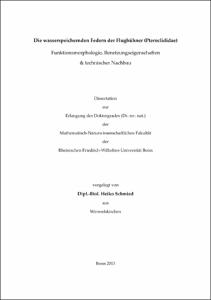This is an image of a scanned piece of white paper with black text, possibly in a different language, making it challenging to decipher. The text appears blurry and is printed in both bold and regular black fonts. The paper is outlined by a thin black rectangle. At the top, there are three rows of black text where the first line is in bold. Below a considerable space, there's a paragraph consisting of a few sentences, with a repetition of a single word three times in the middle. Midway down the page, there are four more lines of text in bold. At the very bottom, two more words are written in black text. The overall layout suggests it could potentially be an invitation or a menu from an upscale establishment.